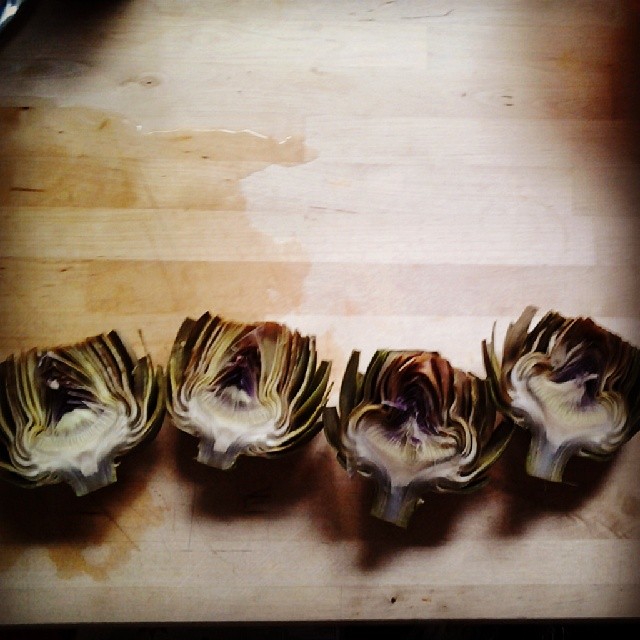A darkly lit photograph showcases a wooden cutting board with a pooled liquid on the left side, imparting a darker yellow hue to the board. At the bottom of the frame, four halved artichokes are arranged side by side, stems pointing downward. The artichokes display a mix of greens and purples with an off-white interior near the stem, revealing their layered structure. The detailed textures and colors of the artichokes contrast against the light brown cutting board, adding depth to the composition.